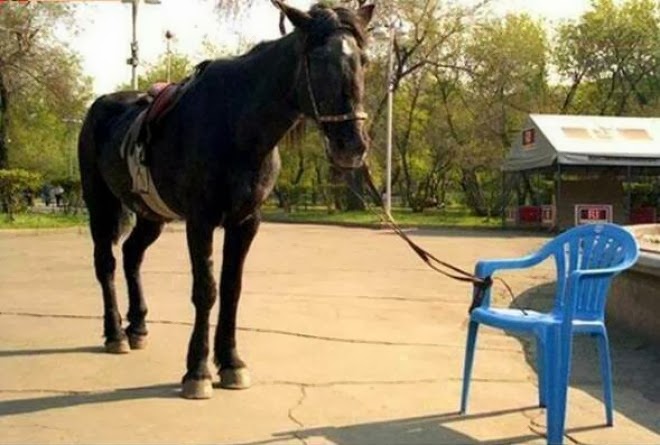In this amusing photo, a tall, mature brown horse stands calmly in a vast, open area bathed in bright sunlight. Adorned with a saddle strapped to its body and reins around its head, the horse’s most striking feature is its mane, which is neatly parted down the middle, revealing two small ears sticking up. What adds to the humor of the image is the unlikely sight of the horse being tethered to a flimsy blue plastic chair, presumably attempting to keep it in place. The backdrop features lush green trees, a small housing tent, and possibly a box marked with "RF." Adding to the scene, two people are visible walking in the distance. The entire setting is lively and vibrant, resonating with the warmth of a sunny day.